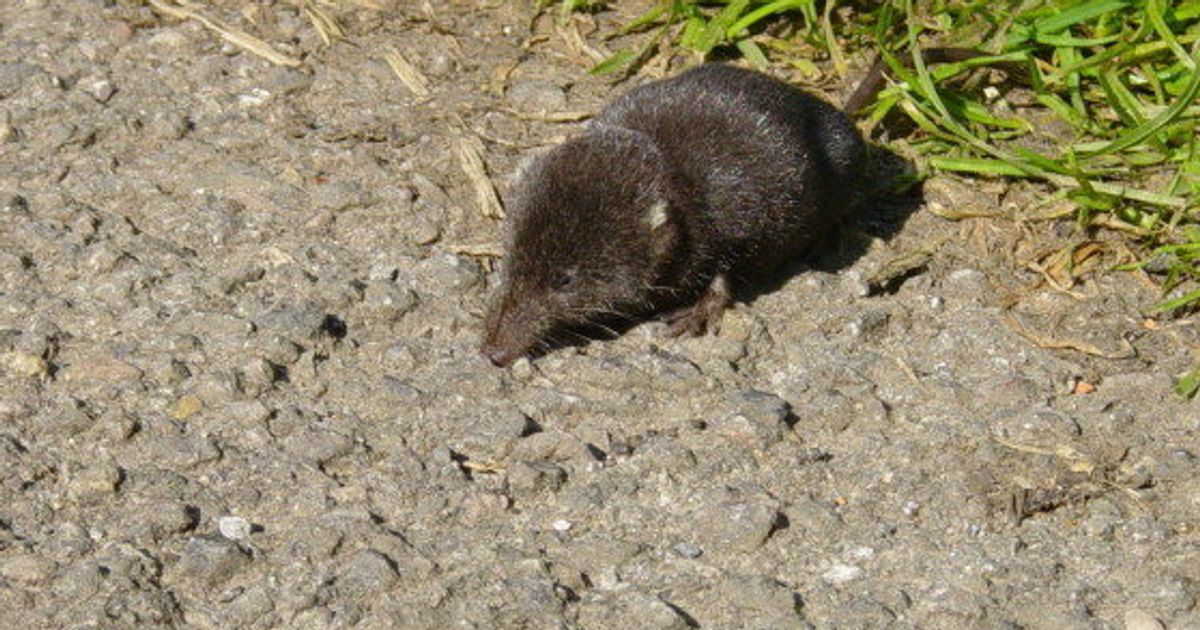The image depicts a small, dark brown rodent-like creature with a long, hairless tail and a pointed snout, resembling a baby mouse, an aardvark, or possibly a vole. This furry rodent is facing slightly left and downward, its front left foot with five small fingers visibly outstretched. It is standing on a flat, dry, rocky terrain covered with gray, tan, and specks of white gravel. Scattered about are some dead weeds, accentuating the rugged surface. In the upper right corner of the image, there is a small patch of light green grass laid down, providing a slight contrast to the otherwise gray and brown setting. Thin white whiskers sprout from the creature's nose, and its long, thin tail stretches towards the green grass behind it.